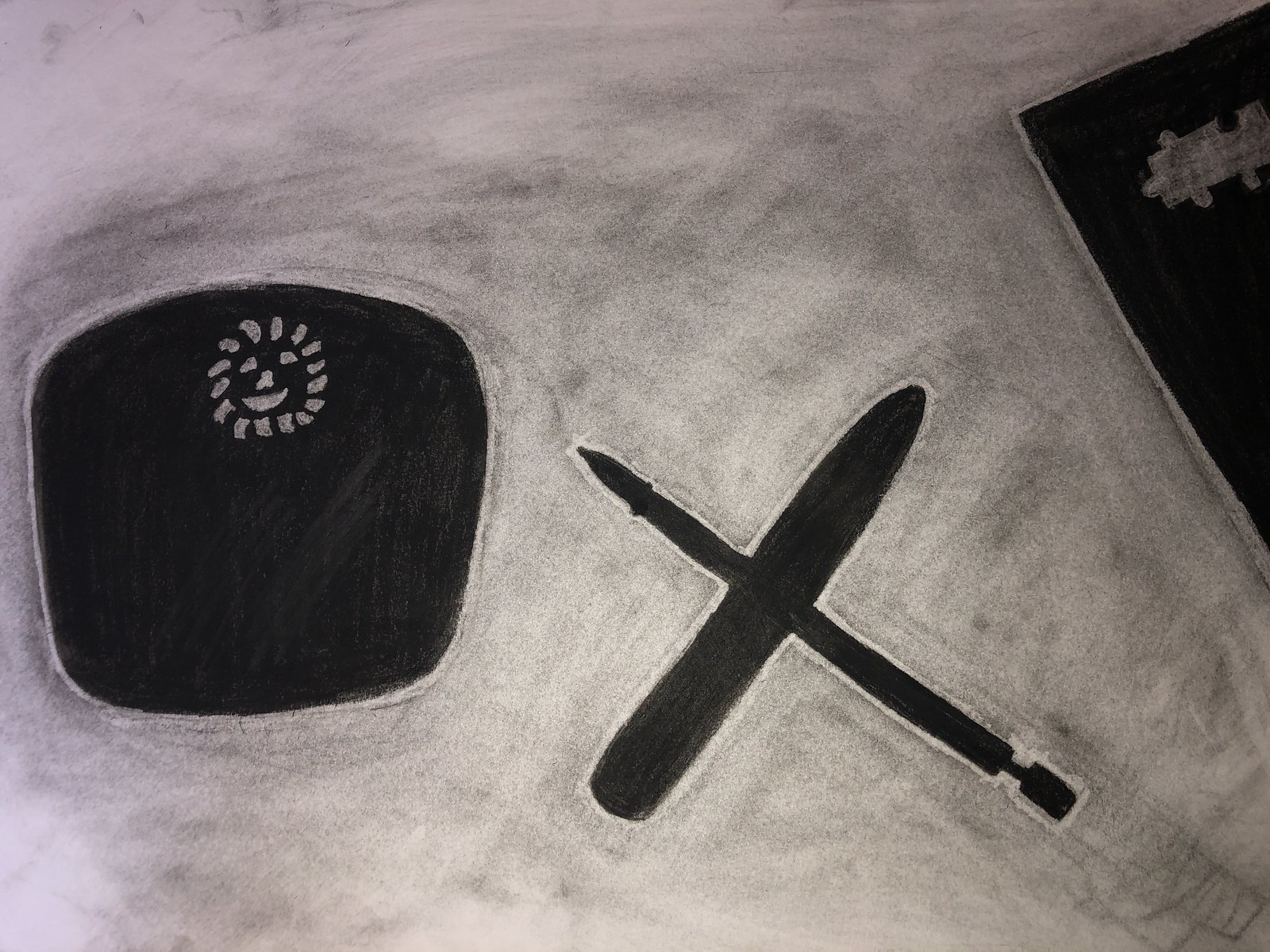The illustration features a white background shaded over with black. On the left side of the image, there is a black rectangle or square that contains a stylized face at its top. This face is defined by two eyes, a nose, and a wide, open smile, surrounded by white curved lines that add a sense of movement or expression. To the right of the square, there is an airplane with its wing prominently extending outward. Within the central part of the image, slightly to the top left, there is an object resembling a cap with an extended brim pointing towards the bottom right. In the top right corner, another black square contains a small white section in the middle and a darker area at the bottom, adding contrast and depth to the overall composition.